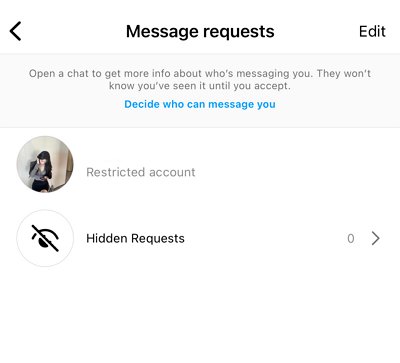This image appears to be a partial screenshot taken from a mobile phone, specifically from an app's messaging interface. The top portion of the screen is visible while the bottom half is cut off, and elements such as the phone's status bar with signal icons are not shown. 

In the upper left-hand corner, a black arrow points to the left, presumably indicating a 'back' function. Centered at the top is the text "MESSAGE REQUEST," bolded and capitalized for emphasis. To the right, there is an option labeled "Edit."

Beneath this header, a gray rectangular box contains informative text. It mentions, "Open a chat to get more info about who is messaging you. They won't know you have seen it until you accept. Decide who can message you," with the latter part highlighted in blue font color.

Further down, the section labeled "Restricted Account" features an image of a person, presumably female, with long, possibly white hair. The individual has their hand up near their face and is wearing black pants or shorts, leaning against what appears to be a wall.

Following that, "Hidden Request" is written alongside an icon of an eye with a line through it, symbolizing hidden or unseen requests. To the right of this section, there is a numeral zero next to an arrow pointing to the right, indicating the absence of hidden requests.